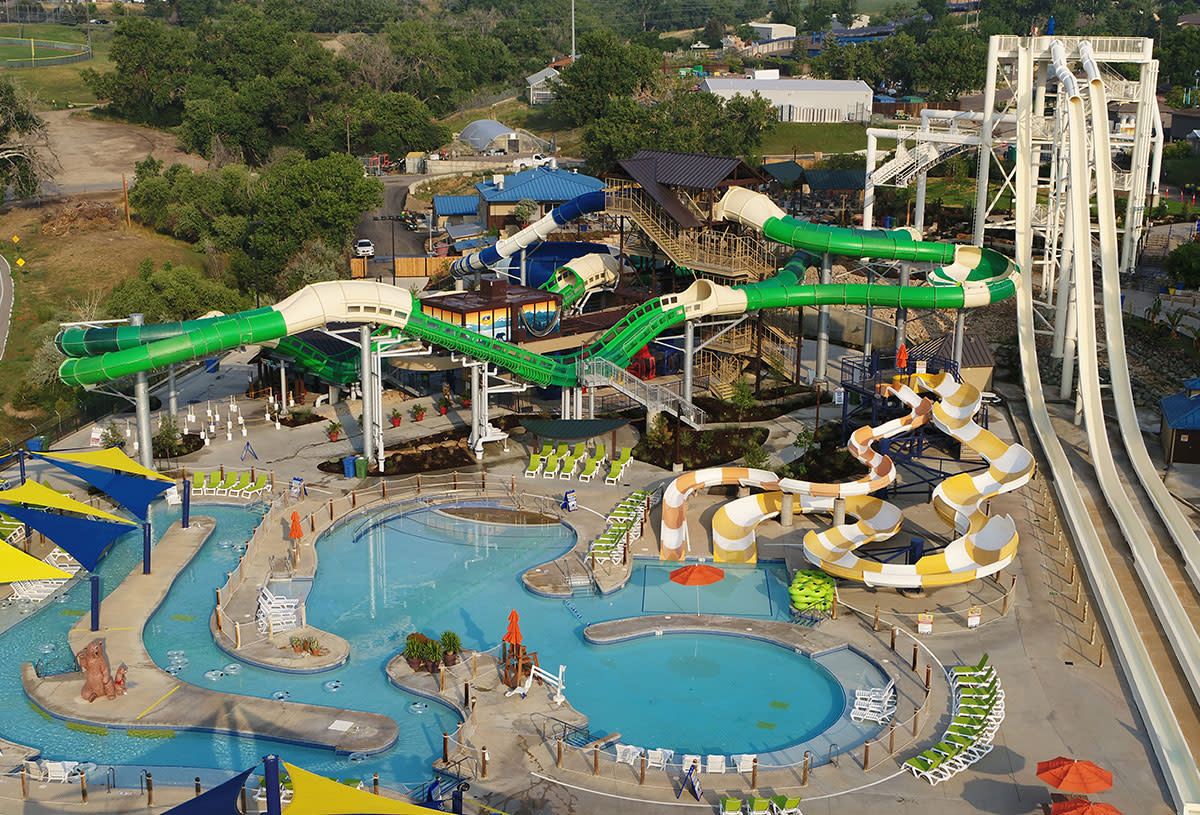An aerial photograph captures an expansive amusement park, with a significant focus on its water park section. Dominating the bottom left corner is a sprawling, irregularly shaped pool, defined by concrete contours that form various sections. This includes two round zones and a squared area where dual yellow and white striped water slides converge. Surrounding the pool are numerous lounge chairs in both white and green, accompanied by three umbrella posts, with one umbrella open and the others closed. 

The right side of the image showcases tall, white water slides, currently devoid of any visitors or visible water flow. In the background, a green roller coaster with contrasting white segments snakes through the park, indicative of its thrilling ride. Further back, another tube, blue with white sections, comes into view, flanked by alternating blue and brown rooftops.

The amusement park is nestled amongst undulating hills with verdant trees, set against a backdrop typical of a village or suburban town, featuring valleys and open spaces. The entire scene is devoid of people, giving an eerie yet serene atmosphere to the park, with the water in the pool shimmering under the light but no signs of activity.